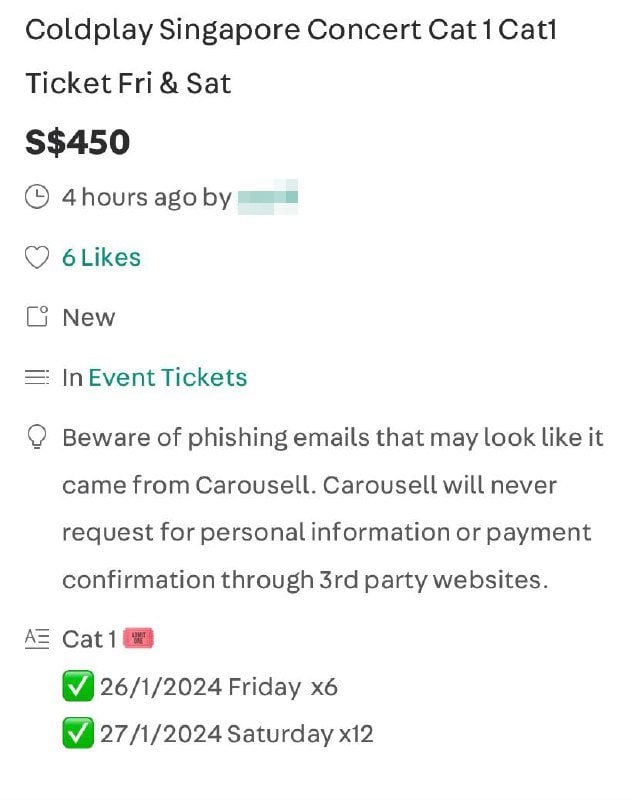The image appears to be a vertically oriented screenshot on a white background. At the top, in black text, it reads: "Coldplay Singapore Concert Cat One Cat One Ticket Friday and Saturday". The first instance of "Cat One" is spaced out with specific separation between "Cat", "T", and "One", whereas the second "Cat One" is written without spacing.

Below this, in a large and bold black font, the price is displayed as "S$450". The image resolution is not very high, resulting in a slight graininess, but the text remains legible.

Further down, it is noted that the post was made "four hours ago" by a user whose name is pixelated, accompanied by a clock icon. Underneath, there is a heart icon and the post has received six likes, which are indicated in blue text. Additionally, there is a "New" label next to the likes.

In the top right-hand corner, there is an icon depicting a square and a small circle, aligning next to the label "Event Tickets" in blue text, which is followed by three horizontal lines.

The bottom section of the screenshot contains a warning message: "Beware of phishing emails that may look like they came from Carousell. Carousell will never request personal information or payment confirmation to third-party websites."

Finally, it states "Cat One" again, denoted by a small pink ticket icon with a checkmark, and lists the concert dates and times as follows: "26/1/2024 Friday 6:00 PM" and "27/1/2024 Saturday 12:00 PM".